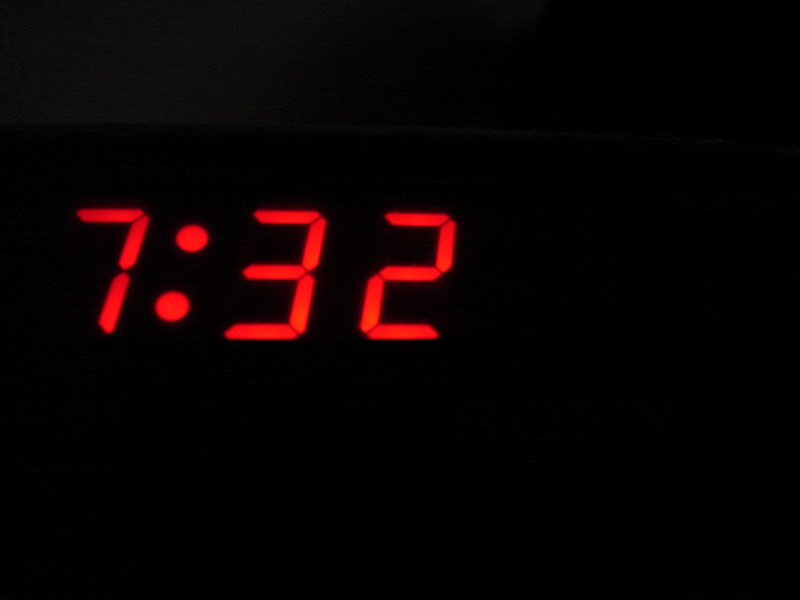The image showcases a stark black square serving as the backdrop. Prominently displayed in the center are the numerals "732," rendered in a vivid red. The numbers are stylized to resemble those found on a digital alarm clock. The simplicity of the composition, with just the bright red digits contrasting against the entirely black background, creates a striking visual impact.